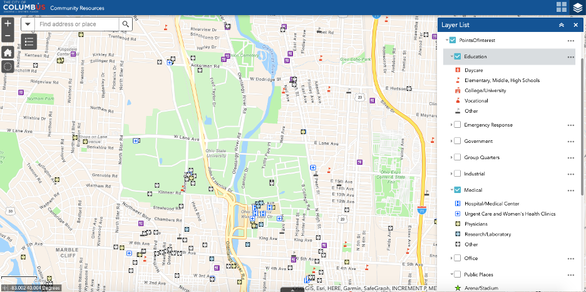The image depicts a digital interface of an app or website, presumably designed for exploring the Columbia area, as indicated by the text in the upper left corner. The word "COLUMBIA" is stylized with "COLUMB" in white and "IA" in red. A blue bar spans the top of the image. On the right side of this bar, there are two icons or logos.

Central to the image is a detailed map. The map showcases various regions with distinct color schemes: a brownish-beige background, patches of green representing grassy areas, and sandy-brown areas adjacent to the green zones. Yellow lines crisscrossing the map indicate roads, and the names of different areas and sections are clearly labeled.

On the right side of the image, there is a prominent white box titled "Layer List." This box contains an extensive selection of items, presented in a list format, offering additional information and options for the user to explore further.